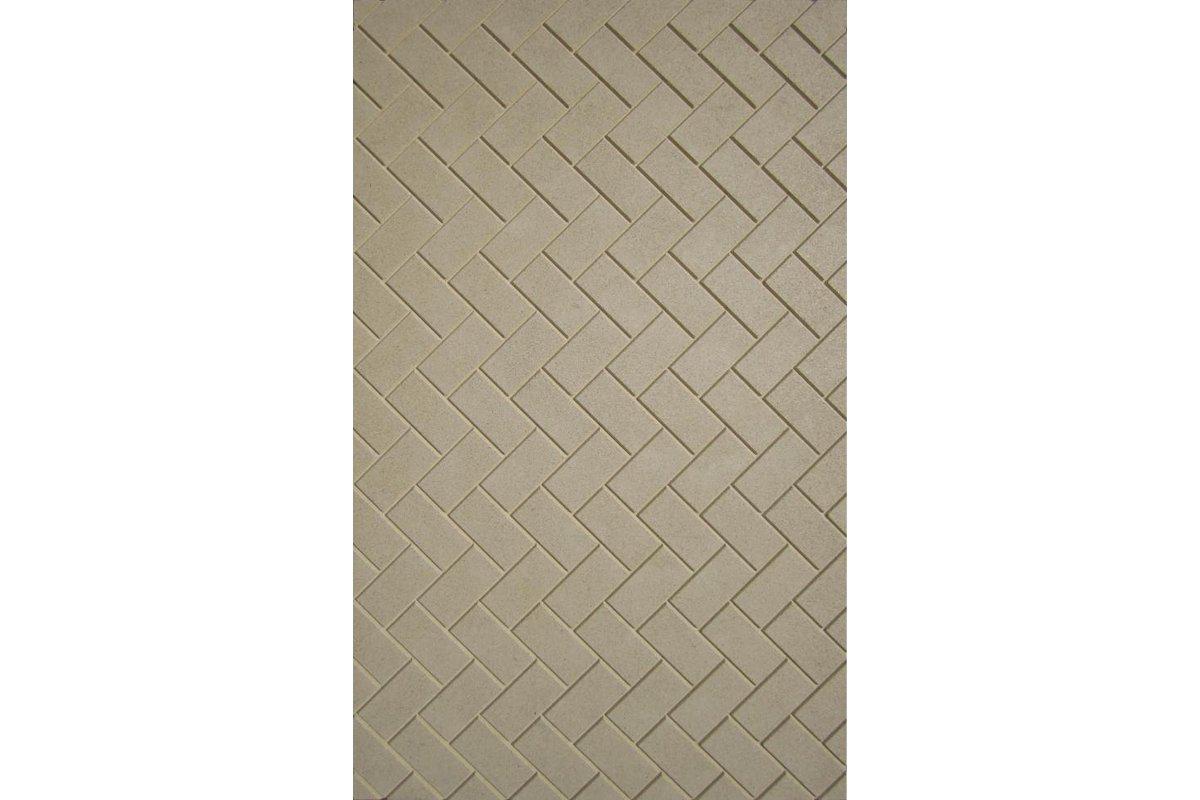The image showcases a detailed and elegant patterned tile surface, characterized by interlocking light beige tiles that form continuous and parallel zigzag patterns. The arrangement of the tiles creates a smooth surface with a sophisticated interlocking design, which alternates between upward-left and upward-right directions, resulting in a striking zigzag effect. The light beige tiles, with slight imperfections and surface dots, provide a distinct and classy appearance that deviates from the more common reddish-brown brick. This intricate pattern extends seamlessly across the surface, emphasizing the refined and uniform look of the tile.